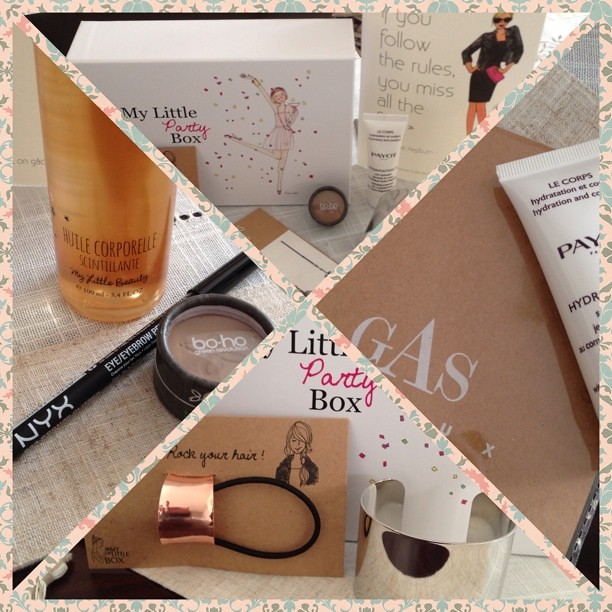The image is a square divided into four triangles by an X, with the borders decorated in a cream color featuring green and pink floral designs. In the top triangle, there's a white box labeled "My Little Party Box" with a cartoon ballerina, surrounded by scattered makeup items and a book titled "If you follow these rules, you'll miss all the fun." The right triangle features a white skincare tube and a darker brown box, partially obscured, with a cartoon woman in a black outfit and sunglasses, holding a pink purse. The bottom triangle showcases two boxes, one being "My Little Party Box" and the other brown box reading "Rock Your Hair," decorated with a cartoon woman. On top are a bronze circular device with a black strap and a silver choker-like accessory. The left triangle includes various cosmetics like a black eyeliner pen labeled "NYX," a black circular makeup package, a white serum bottle with foreign text, and a small cylindrical container marked "Boho." All elements together reveal a coordinated arrangement of beauty products and packaging.